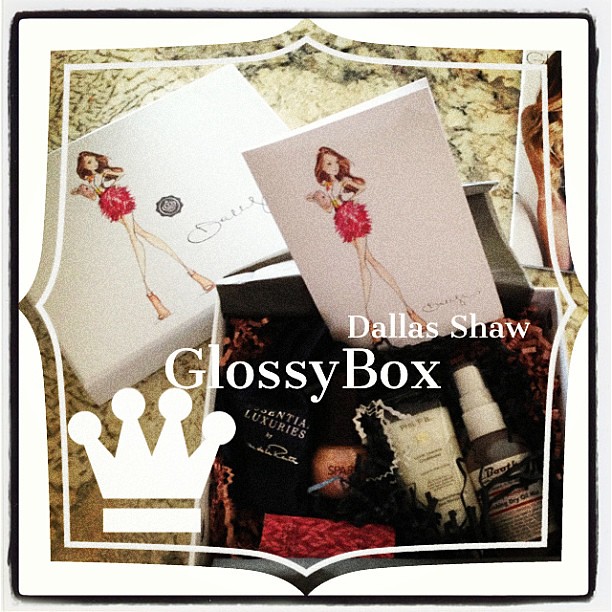The image is a richly detailed advertisement for Dallas Shaw's luxury monthly subscription box, featuring a distinctive box cover adorned with a stylish, leggy cartoon female sporting a fluffy red skirt, long brown hair, and pink high-heeled boots. The depiction of this character, also printed on a card emerging from the box, alongside the prominent "Dallas Shaw Glossy Box" branding, lends a consistent and elegant aesthetic throughout. Encasing the photograph is a fancy black and white frame, a design that complements the white and black marble background on which the open box rests. Within the box, nestled in crinkly beige packing paper, are various beauty and wellness goodies, including a white bottle of cream, a pump spray bottle with a white top, a round container with a red substance, and a black bag labeled "essential luxuries." The lower left corner of the image is marked with a white crown emblem, reinforcing the luxurious theme of the entire presentation.